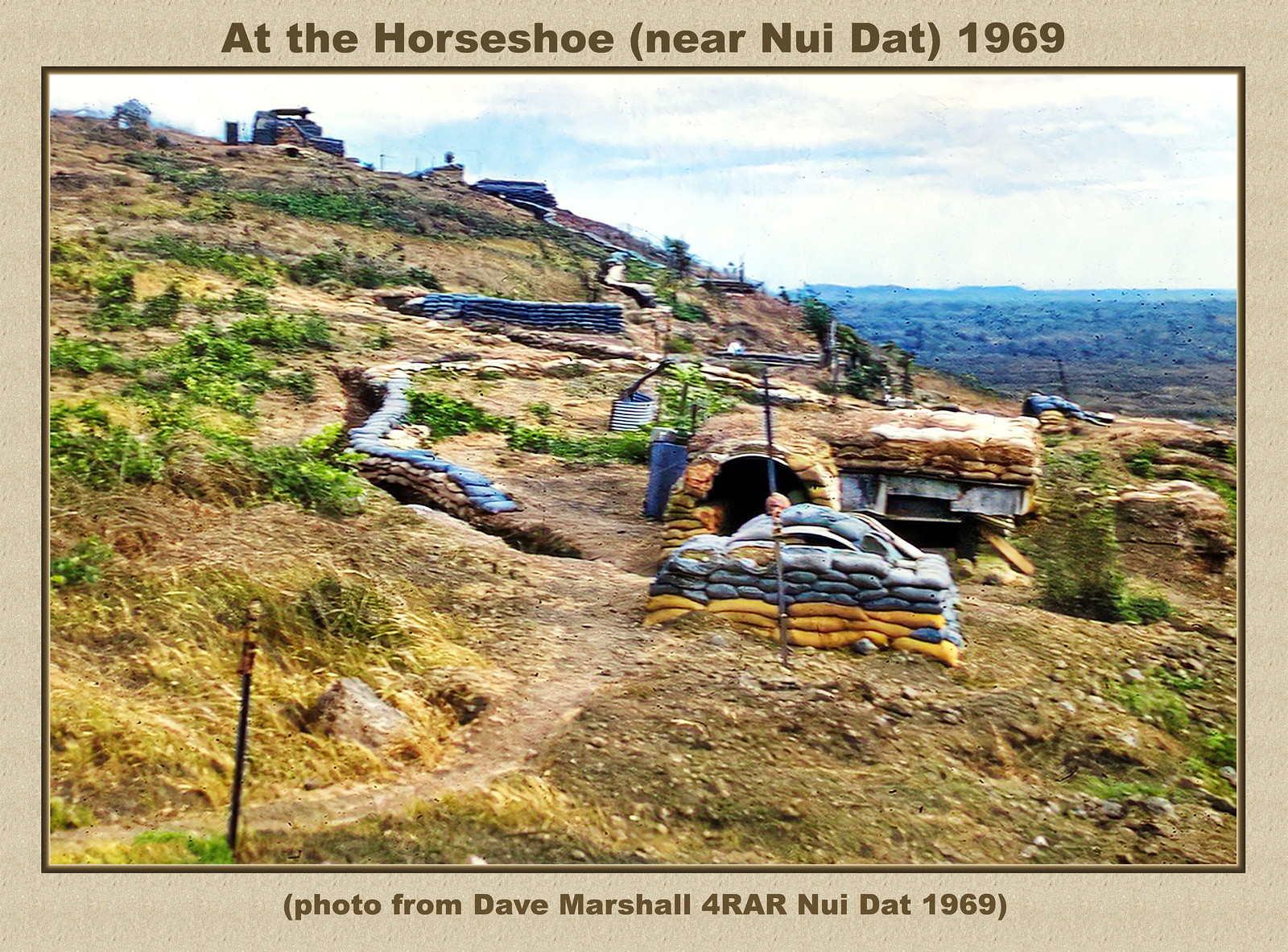In this 1969 photograph captioned "At the Horseshoe near Nui Dat," provided by Dave Marshall for RAR, the scene unfolds on a barren hillside characteristic of the Vietnam conflict era. The image is framed with a tan border featuring brown writing, detailing its historical context at both the top and bottom. The foreground is dominated by a landscape marked by a network of fortified sandbags, some stacked in alternating blue and yellow layers. These sandbags create a defensive structure, including a small tunnel or crawl space, and are likely intended for combat use.

A man peers out from behind the sandbags, observing the camera. The surrounding environment appears damp, with sparse vegetation—occasional green bushes break through the predominantly dark brown dirt and grass. More expansive views extend to the right side of the image, where a broad plain reaches toward a bright, mostly pale blue sky with streaks of darker blue. The hillside itself is textured with brown and green hues, dotted with makeshift huts and further fortifications. Off-center to the left, a trench or foxhole is visible, adding to the scene's somber readiness for conflict.